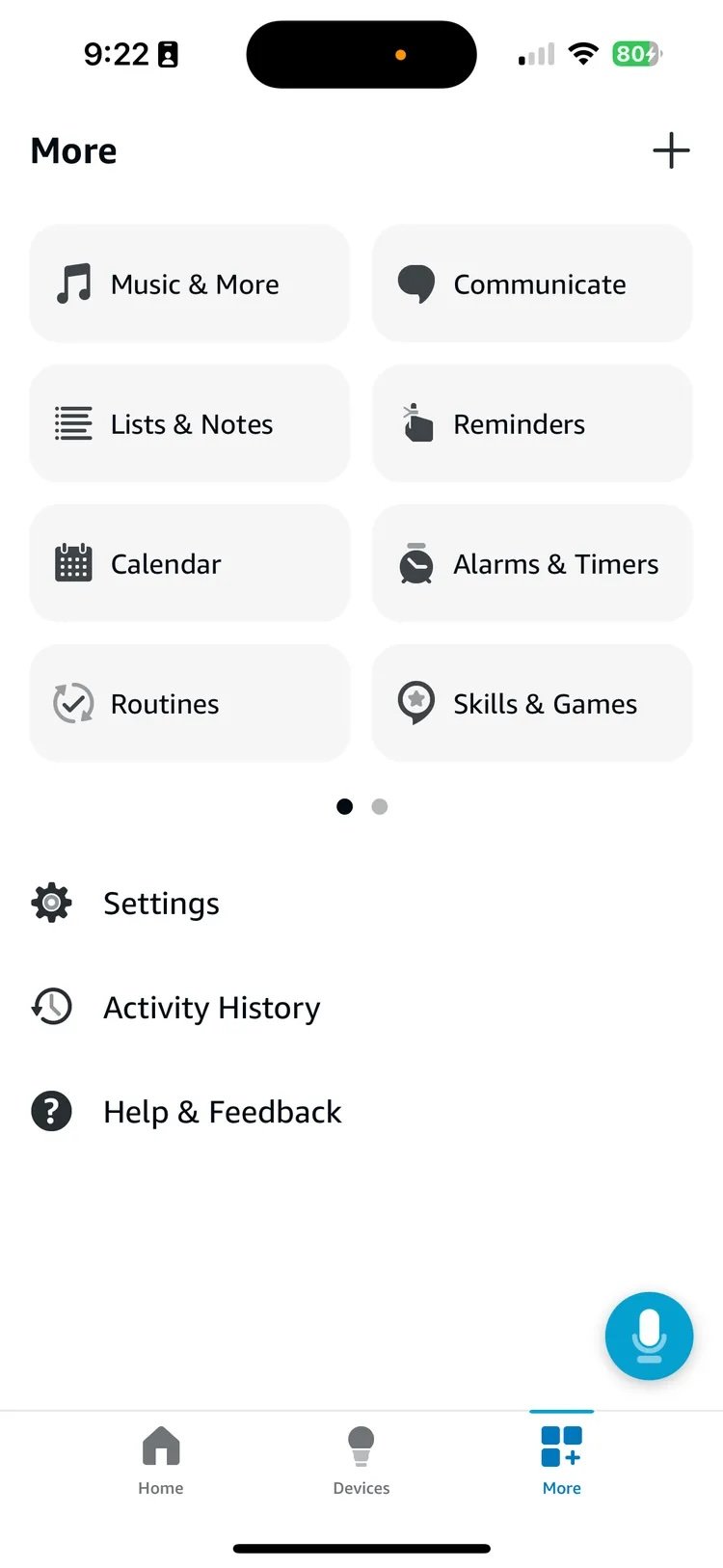In the image depicted, we see a white background resembling a smartphone interface. The top-left corner displays the time as 9:22 AM near a phone icon. To the right, there's a black oval section featuring an orange dot in the center. The Wi-Fi signal indicator is weak, and the battery level is at 80%.

Below this, in black font, the word "MORE" is displayed, accompanied by a plus sign (+) to the right. Just beneath it, there are approximately eight gray circles arranged in two rows. Each circle contains distinct functionalities:

1. The first circle, labeled "MUSIC & MORE," features a music note icon.
2. The second circle, labeled "COMMUNICATE," contains a speech bubble icon.
3. The third circle, labeled "LISTS & NOTES," showcases a lines icon.
4. The fourth circle, labeled "REMINDERS," is located to the right of the previous circle.
5. The fifth circle, labeled "CALENDAR," has a calendar icon on the left.
6. The sixth circle, labeled "ALARMS & TIMERS," includes a clock alarm icon.
7. The seventh circle, labeled "ROUTINES," displays a checkmark within two curved arrows forming a circle.
8. The eighth circle, labeled "SKILLS & GAMES," features a star in the middle of a circle.

At the bottom, we have two distinct shaded dots, one darker and one lighter gray. Below these dots are three sections:

1. "SETTINGS," with a settings gear icon.
2. "ACTIVITY HISTORY," with an arrow looping around a clock.
3. "HELP & FEEDBACK," with a gray circle containing a white question mark.

To the right of these sections, there's a blue circle housing a white microphone icon.

Further down, the interface displays three options beneath a gray line: "HOME" (with a home icon), "DEVICES" (with a light bulb or microphone icon), and "MORE" (with three squares and a plus sign), all in blue font. Lastly, at the very bottom, there is a solid black line spanning the width of the screen.